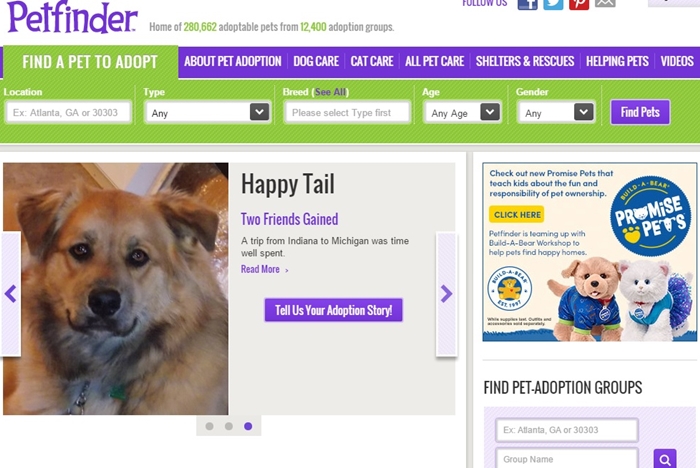A screenshot from a desktop browser displaying the Petfinder website. The Petfinder logo is visible at the top left. The site boasts having 280,662 adoptable pets from 12,400 adoption groups. The top menu features a green background with white text that says "Find a Pet to Adopt." The menu offers search options including location, type, breed, age, and gender, followed by a purple "Find Pet" button. Additional menu options with purple backgrounds include "About Pet Adoption," "Dog Care," "Cat Care," "All Pet Care," "Shelters and Rescues," "Helping Pets," and "Videos."

Below this menu, there is an article featuring an image of a dog on the left with a headline titled "Happy Tail: Two friends' trip from Indiana to Michigan was time well spent." There's an invitation to "Read More" and a purple "Tell Us Your Adoption Story" button. Users can scroll horizontally through stories. On the right side, an ad promoting "Promise Pets" is visible. Further down, there is information on finding pet adoption groups.